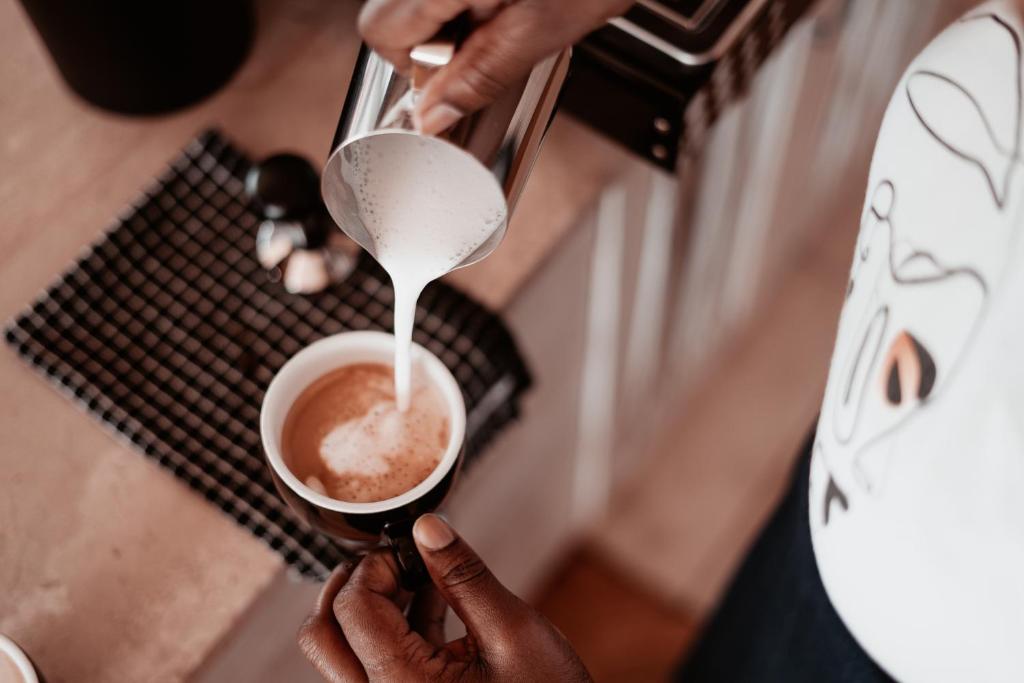In this detailed, horizontally rectangular color photograph, likely taken indoors with artificial light, a dark-skinned woman's hand is visible from an overhead viewpoint, pouring white cream from a small, silver chrome pitcher into a black coffee cup. The black coffee cup has a white interior and is held steady by her other hand, gracefully displaying three fingers grasping it. The image captures the action clearly, making it a staged snapshot of a serene moment. The coffee and cream sit atop a brown, wooden countertop, and in the blurred background, you can spot white cabinets and a checkerboard patterned towel. The woman's attire is a simple white t-shirt adorned with a minor black design, suggesting a casual yet intentional setup. The meticulous composition of the photograph emphasizes the contrast between the rich hues of the coffee and the creamy swirl being created, framed by the subtleties of everyday kitchen elements.